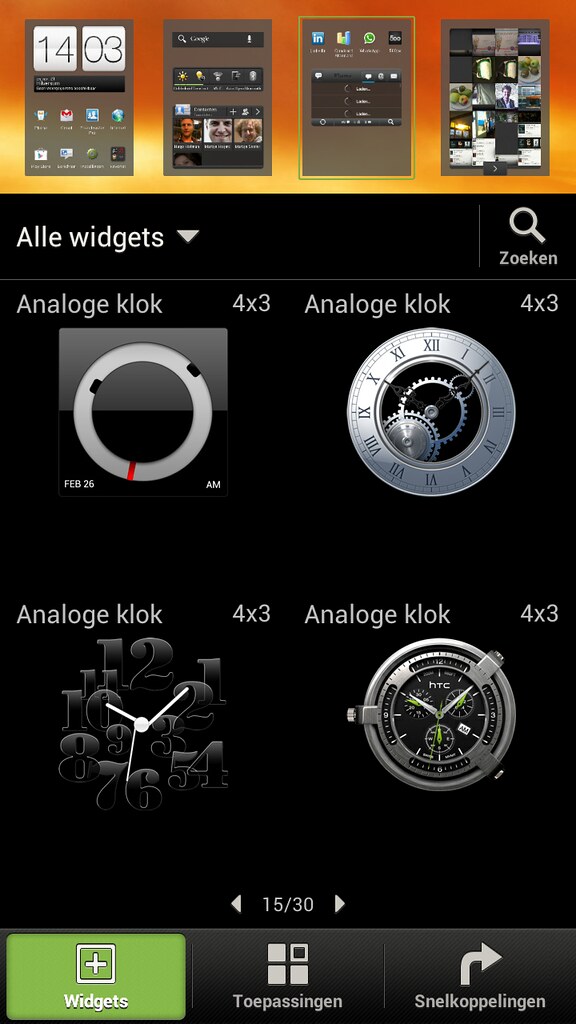The image is a screenshot from a phone showcasing a multi-panel interface. The top section features a gradient in orange, yellow, and white, containing four smaller panels. From left to right, these panels display: the time, '14:03', along with some app icons; a search bar overlapping more app icons and files; another assortment of icons and images; and a section appearing to be a camera roll with several images. Below this top section, the main central portion of the screenshot has a black background with the title "ALE Widgets" at the top, followed by a down arrow. Directly underneath, there are various entries labeled "analog cloak" repeated multiple times, seemingly different versions or themes available. At the extreme bottom of the image, there are three buttons. The left button, labeled "Widgets," is in green. The middle button is labeled "Topasingan" and features four square icons. The right button, whose label could not be fully discerned, features an arrow pointing to the right. The overall layout suggests navigable widgets and settings, highlighting a detailed interface with multiple functionalities.